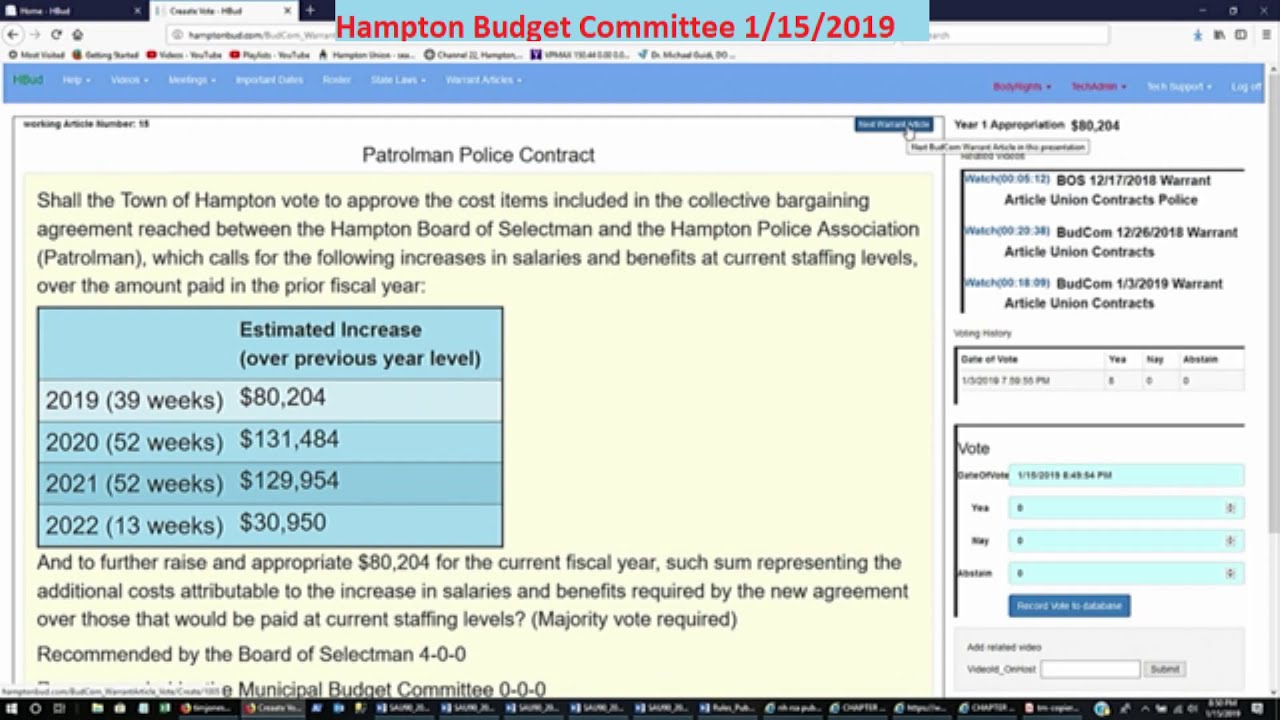The image is a webpage screenshot detailing a budget referendum for the Town of Hampton, prominently showing the date "Hampton Budget Committee 1-15-2019" in red letters at the top. Beneath this, there is a blue navigation bar featuring various menu options. The main portion of the screen showcases a section titled "Patrolman Police Contract." The highlighted text on a yellow background reads, "Shall the Town of Hampton vote to approve the cost items included in the collective bargaining agreement reached between the Hampton Board of Selectmen and the Hampton Police Association Patrolman, which calls for the following increases in salaries and benefits at current staffing levels over the amount paid in the previous fiscal years." This section also includes a projected four-year financial outlook and specifies that the proposed increase is $80,000 for the current fiscal year. Additional details indicate "recommended by the Board of Selectmen 400" and "municipal budget committee 000," emphasizing that a majority vote is required. On the right-hand side, there's an interface possibly related to voting on the budget or modifying projections. The primary colors used in the image are yellow, blue, and white.